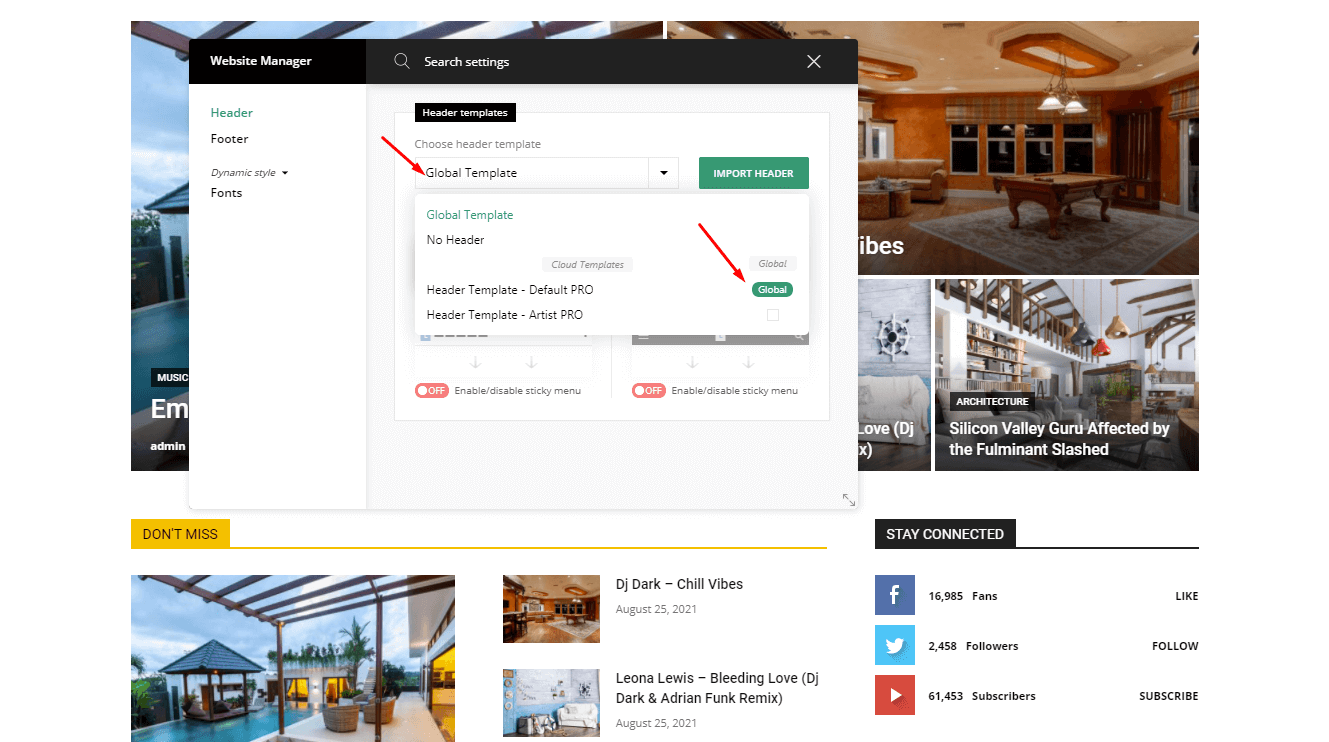The image appears to be from a real estate or rental website, possibly showcasing properties such as homes, condos, or hotels. It features an array of appealing photographs, including stylish homes, inviting patios, and luxurious pools. However, a dialog box is prominently positioned in the center of the screen, obscuring details about the properties and any pertinent information. On the right side, there are links to social media platforms for staying connected, including Facebook, Twitter, and YouTube. At the bottom, a section labeled "Don't Miss" seems to highlight special deals or opportunities available for purchase or lease.